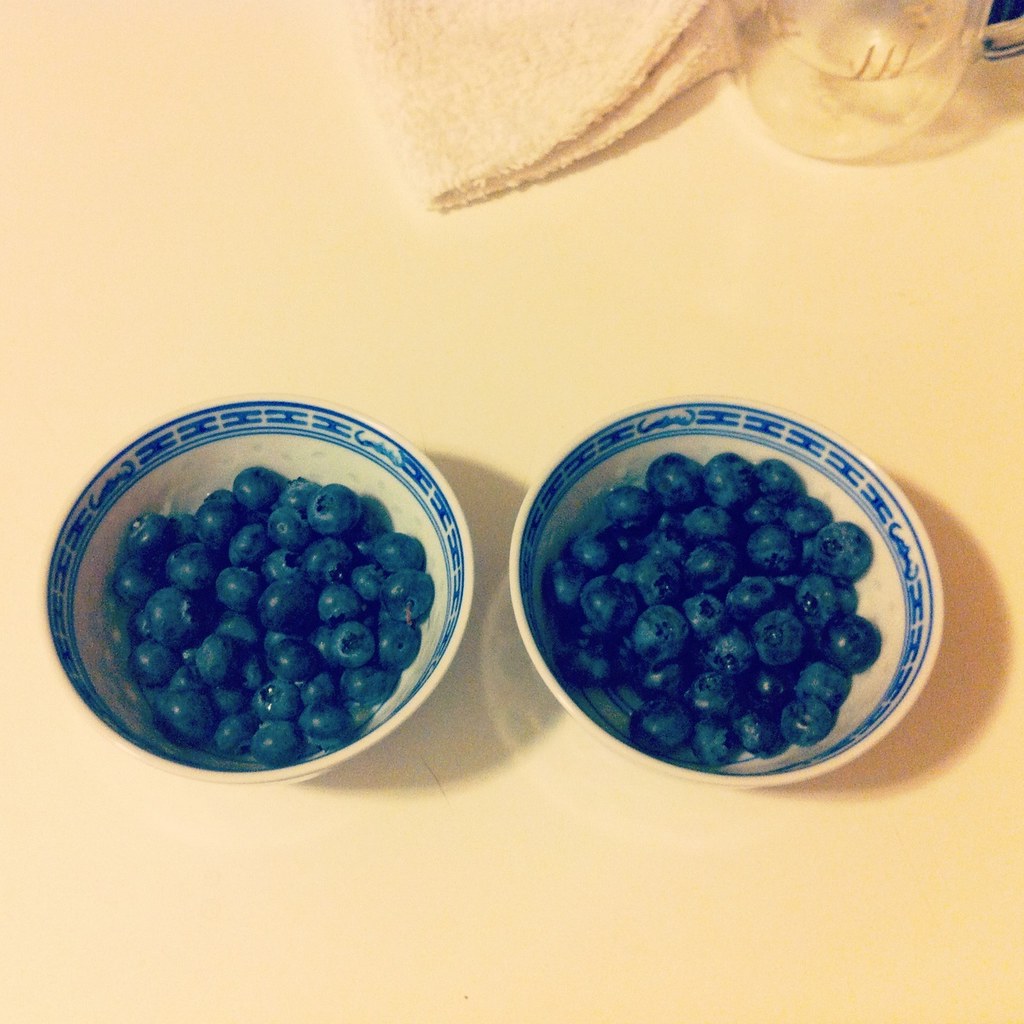The image features two white bowls with a blue patterned trim containing fresh blueberries, sitting side-by-side on a tan, orangish tablecloth or surface. The trim on the bowls includes blue squares, circles, and sideways-looking H's and measures about half an inch in comparison to the blueberries. Each bowl is filled to approximately two-thirds to three-quarters full, with one appearing slightly fuller than the other. In the upper portion of the image, there is a partially visible clear glass or jar with a clear liquid, possibly water, and a handle. Adjacent to the glass is a neatly folded dishcloth or napkin in the same tan color as the tablecloth. The overall setting places the focus on the two bowls of vibrant, juicy blueberries.